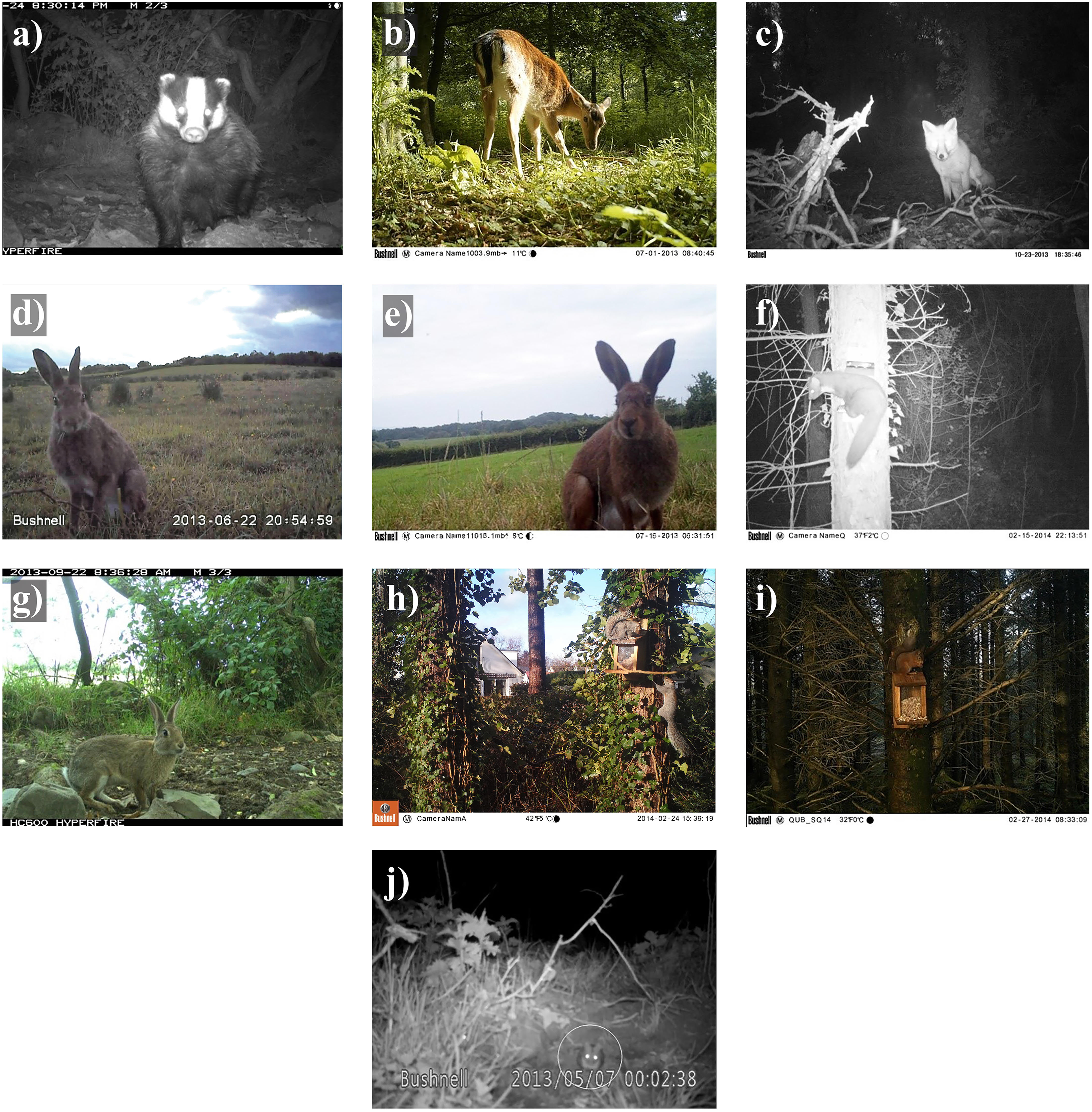The image is a detailed collage of 10 trail camera photographs arranged in a grid format of three rows with three images each, and one at the bottom. Each photograph is labeled alphabetically from A to J with bold white Times New Roman lowercase letters. These appear to be captured by a wildlife camera, as indicated by the visible time stamps from 2013 and 2014. 

- **A** features a black and white shot of a badger, captured at night.
- **B** shows a deer, specifically a fawn, in daylight.
- **C** presents a fox photographed in night vision.
- **D** and **E** both depict rabbits during the day.
- **F** captures what looks like a tree-climbing shrew or ferret at night.
- **G** includes another daytime rabbit.
- **H** and **I** both involve squirrels; one is shown near what appears to be a bird’s nest or feeder, possibly with seeds.
- **J** shows a small animal, potentially a mouse or muskrat, in night vision, though it’s small and a bit unclear.

Each photograph authentically captures a moment in the wildlife environment, showcasing a variety of animals in their natural habitat.